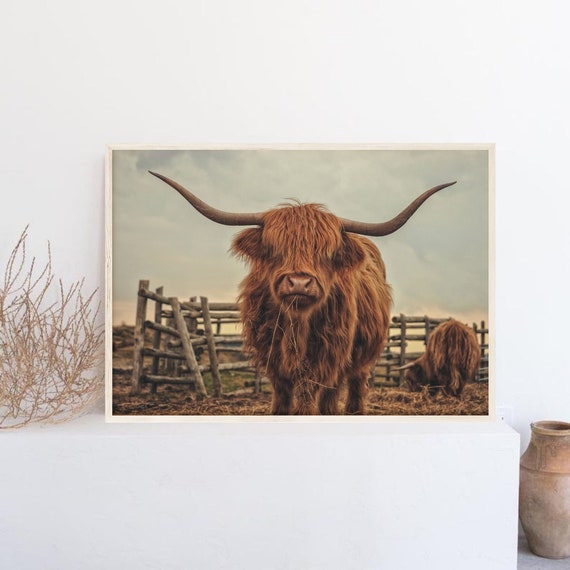This is a detailed decorative home photo displayed against a white wall. The picture is framed in a thin, white wooden frame, with some conversation noting a beige tint to the border. The image itself is a high-resolution photograph depicting a brown, fuzzy Highland cow with long, turned-up horns, its face obscured by thick hair, showcasing only its nose and mouth. Behind it is a wooden picket fence, and to the right in the background, another Highland cow is munching on some hay. The background features a cloudy, overcast sky. The white counter, acting as a base for the frame, merges seamlessly with the white wall. To the left of the frame sits a decorative dried tumbleweed or light brown branches, adding a rustic touch. Below on the right on the floor is a light brown clay pot or vase, standing almost parallel to the counter shelf. This arrangement creates a harmonious and detailed aesthetic, perfect for home decoration.